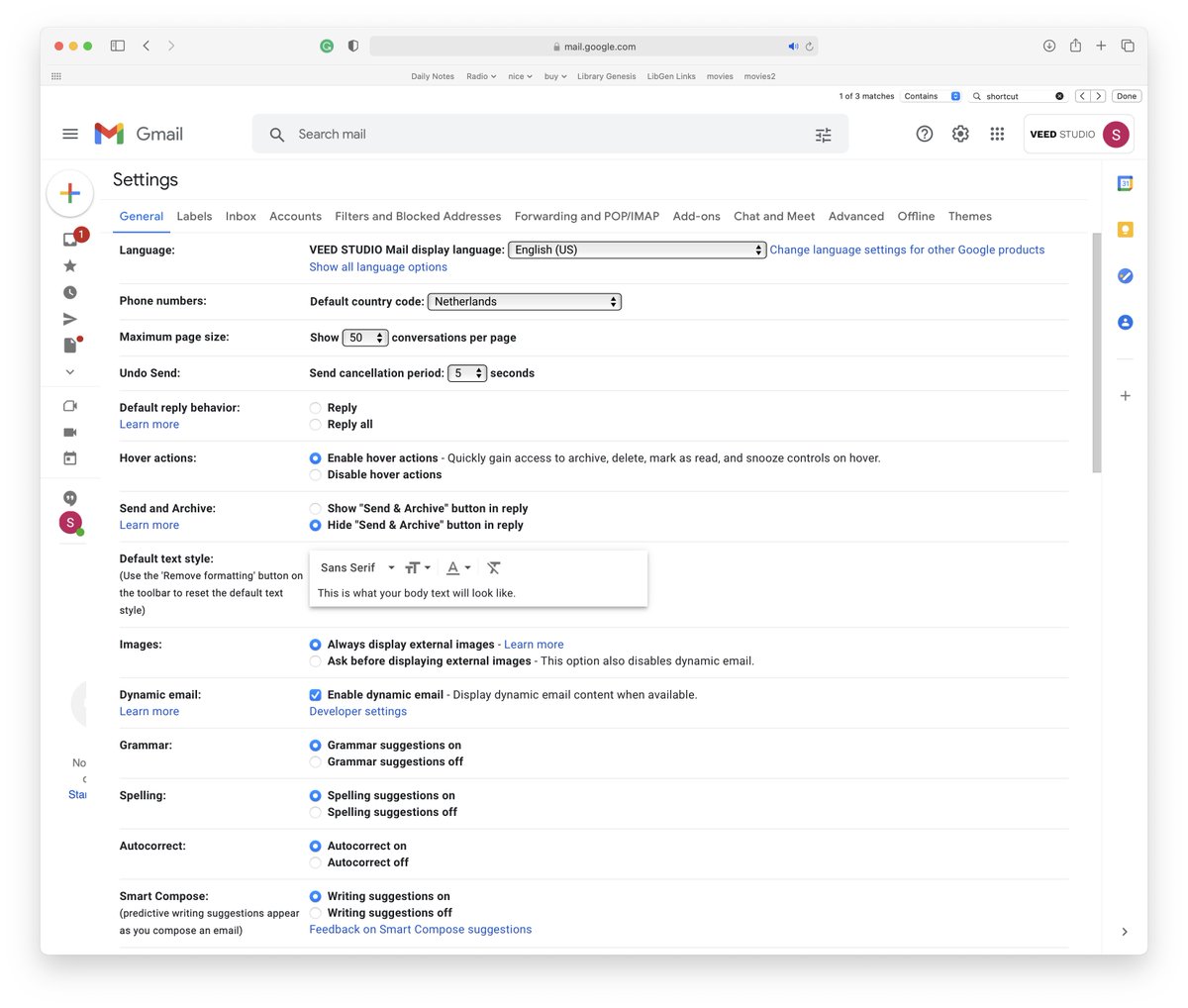This screenshot depicts the settings interface of Gmail's website. In the top-left corner, the recognizable Gmail logo is visible, displaying its characteristic multicolored "M" in shades of blue, red, yellow, and green. The interface indicates that the user is currently within the settings section of Gmail, as "Settings" is prominently displayed below the logo. 

The settings are organized into a plethora of tabs, arrayed from left to right, including: General, Labels, Inbox, Accounts, Filters and Blocked Addresses, Forwarding and POP/IMAP, Add-ons, Chat and Meet, Advanced, Offline, and Themes. The "General" tab is visibly selected, highlighted in blue with a blue underline distinguishing it from the others.

Beneath these tabs, several specific settings are listed. Notable entries include options for adjusting language preferences, phone numbers, maximum page size (set to 50 conversations per page), undo send duration, default reply behavior, never actions, send and archive, and the default text style, which is set to sans-serif.